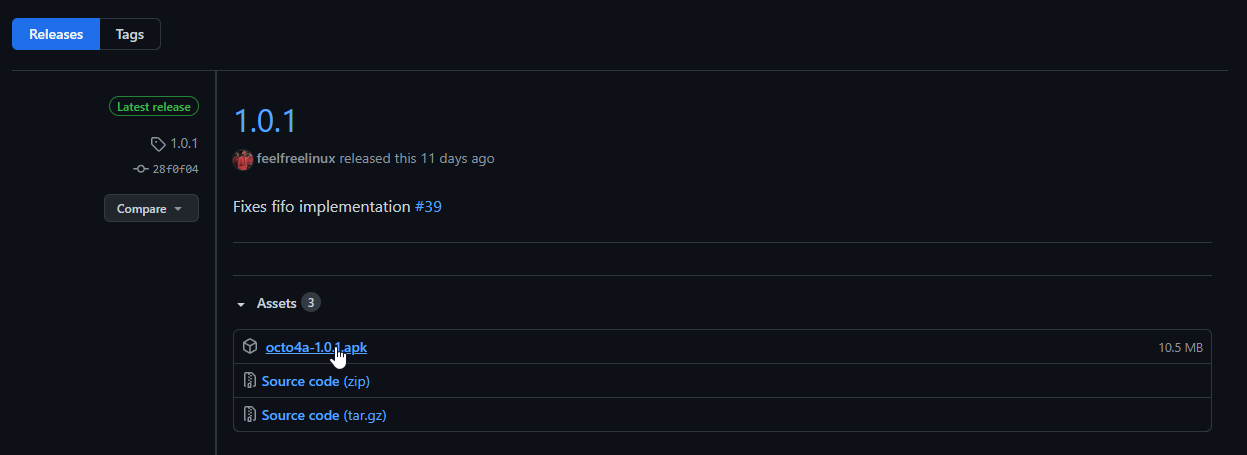Here we have an image of an information update on a website or app, viewed in a dark mode setting with a black background. 

In the upper left corner, there are two interactive buttons: "Releases" and "Tags." The "Releases" button is highlighted in blue, indicating that the user is currently on this page, while the "Tags" button blends into the black background.

Directly below these buttons is a thin gray line, both horizontally and vertically. To the left of this line, it states "Latest Release 1.0.1" in green, followed by the identifier "28F0F04" and a "Compare" dropdown menu.

On the right side of this section, it again mentions "1.0.1" in blue text, accompanied by the message "Free Feel Free Linux released this 11 days ago." Below this, it notes the fix "Fixes FIFO inflammation number 39."

At the bottom, there are three listed assets available for download:
1. Octo 4a dash 1.0.1 APK
2. Source code (zip)
3. Source code (tar.gz)